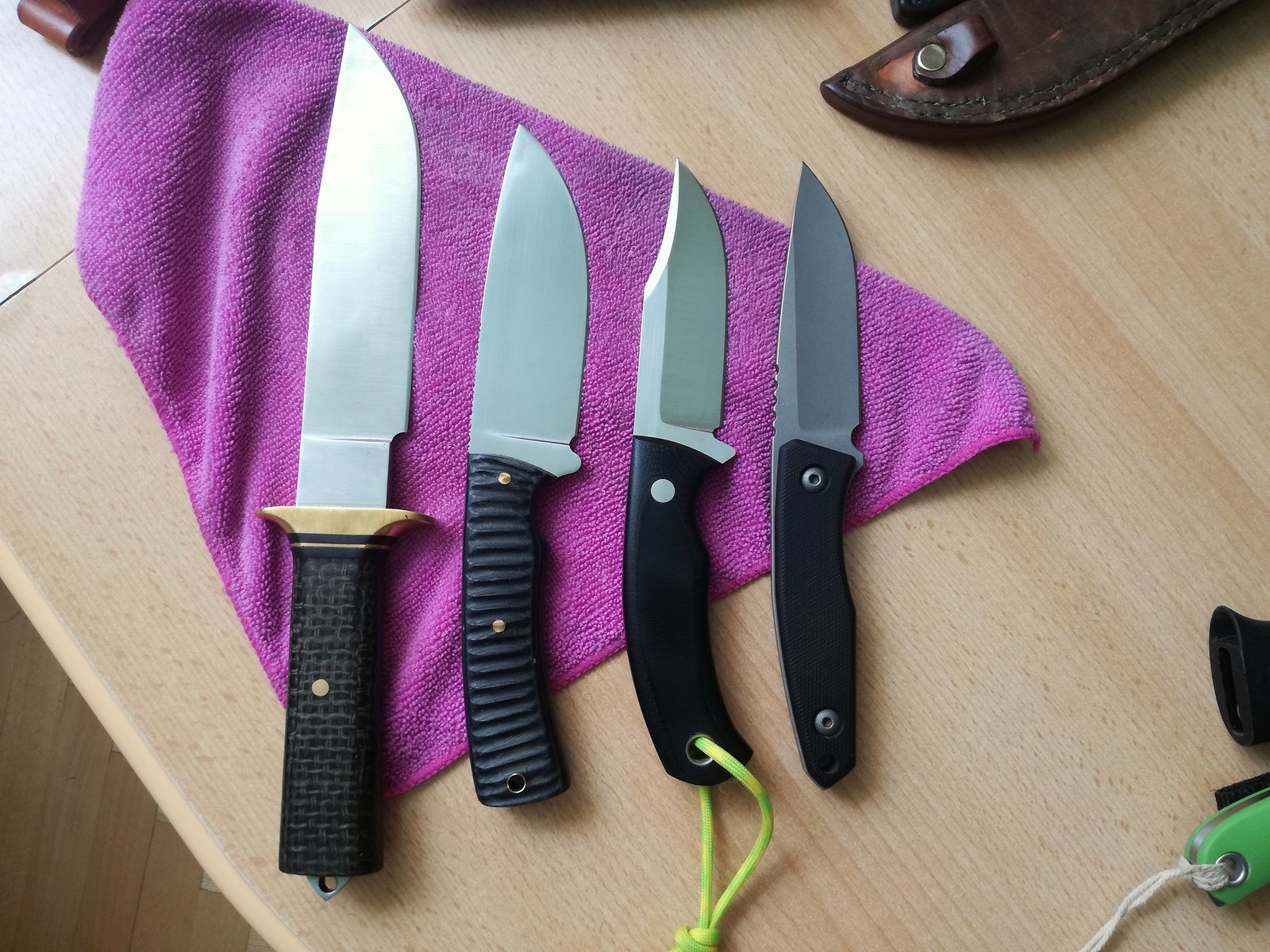In the photograph, a blonde wooden table serves as the base for a carefully arranged setup. The table's natural wood tone contrasts slightly with the darker wooden flooring beneath it. On top of the table, a pink (almost purple) towel has been folded into a triangular shape, with the tip of the triangle pointing towards the bottom left corner of the image. Arranged neatly on this towel are four hunting knives, each with distinctive designs and black handles. 

Starting from the left side, the first knife features a black handle embedded with gold-colored accents. The second knife to its right also has a black handle but is distinguished by textured lines and golden pieces securing the handle together. Moving further right, the third knife boasts a black handle with a silver tip and a silver pin holding it together. It also has a green and yellow string looped through a hole in the handle. The fourth knife, located towards the bottom right of the towel, has a black handle with two gray screws. One can see a faint white string emerging from part of this knife's end.

In the bottom right corner of the image, you can identify part of a handle that includes a hole and has white and green strings hanging from it. The top right corner of the image features a brown leather sheath with double stitching and a silver nail securing it, presumably for one of the knives. The lighting and orientation provide a comprehensive view of the items, highlighting the contrast between the natural wood, the colorful towel, and the metallic sheen of the knives' blades.